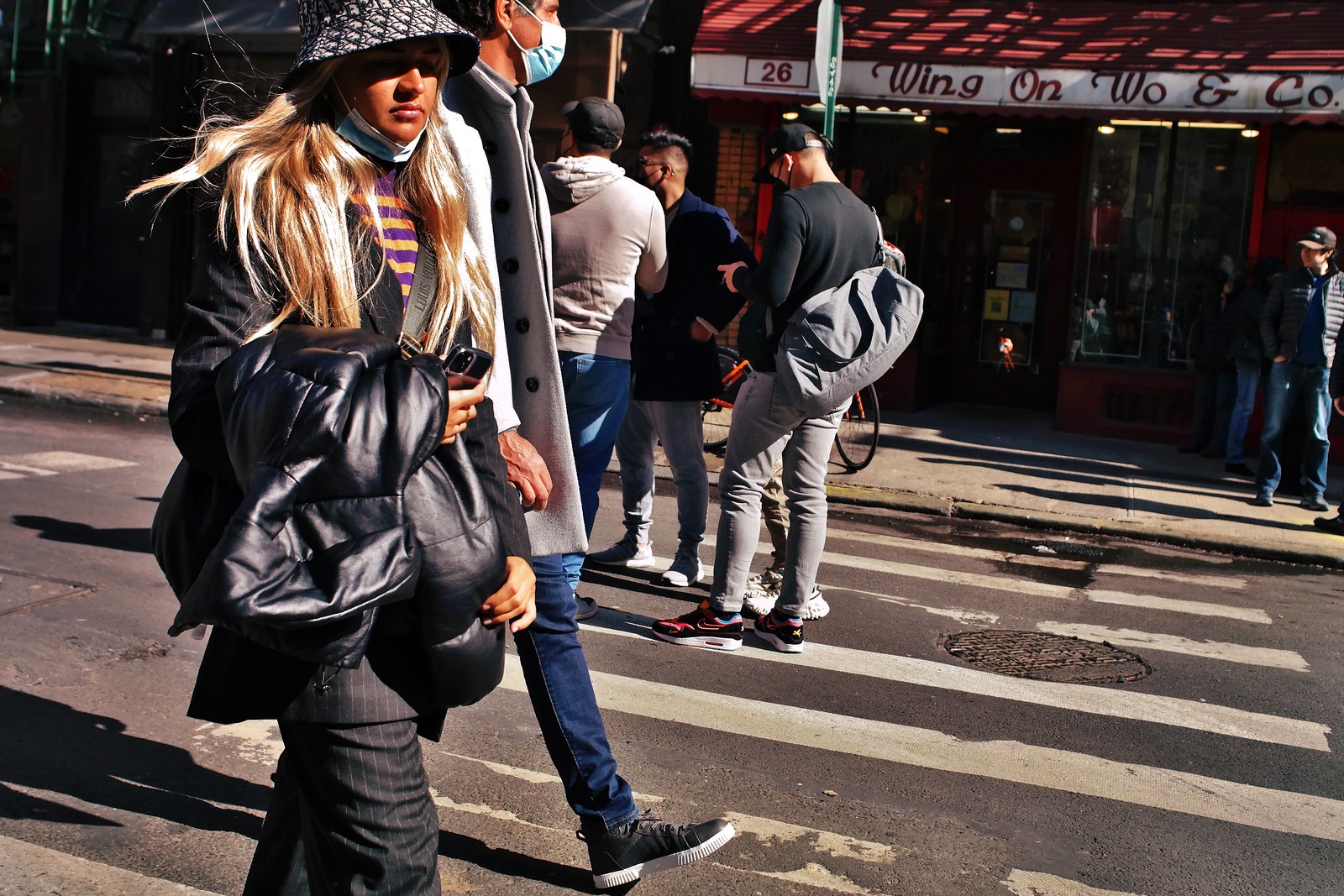The photograph is an urban street scene featuring several people and buildings. In the foreground, a woman with long blonde hair, wearing a patterned bucket hat and a PPE mask around her neck, holds a jacket and her phone. She is dressed in a black jacket, purple and gold striped shirt, black pants, and pinstripe pants. Next to her stands a man in a gray winter coat, blue jeans, and black shoes with white soles, sporting a light blue medical mask over his face. 

In the middle of the street, four young men congregate in a small group, all wearing PPE masks and some looking at their phones. There are also two people walking on the street, adding to the bustling atmosphere. 

The backdrop includes buildings lining the street, and a specific storefront catches the eye with a red awning and a white section bearing the name "Wing On Woe and Co." The detailed and lively urban scene is set against a background of typical corner stores and city architecture, suggesting a cold weather season with people dressed accordingly.